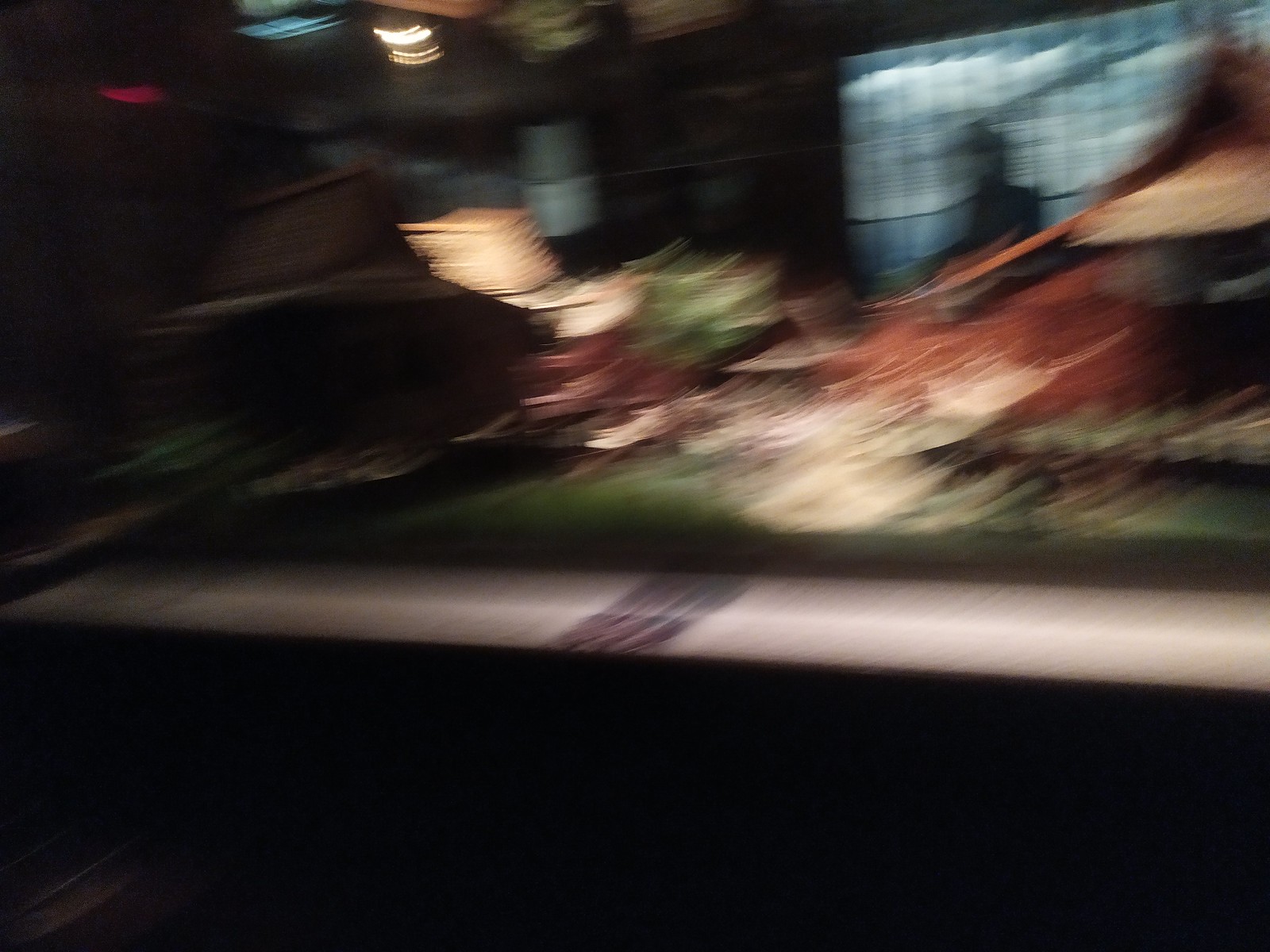This is an intensely motion-blurred photograph depicting a dimly lit room. Central in the frame is what appears to be a chair, albeit obscured by the blurriness. The floor is covered with a greenish rug and seems slightly elevated, suggesting the scene might be set on a platform—possibly indicating it's a stage or a display area, such as one found at a home and garden show. To the right of the image, there's a window emitting some light through partially visible blue sheer drapes, behind which a dark figure is faintly discernible. Overhead, several lights are visible, casting faint illumination across the setting.